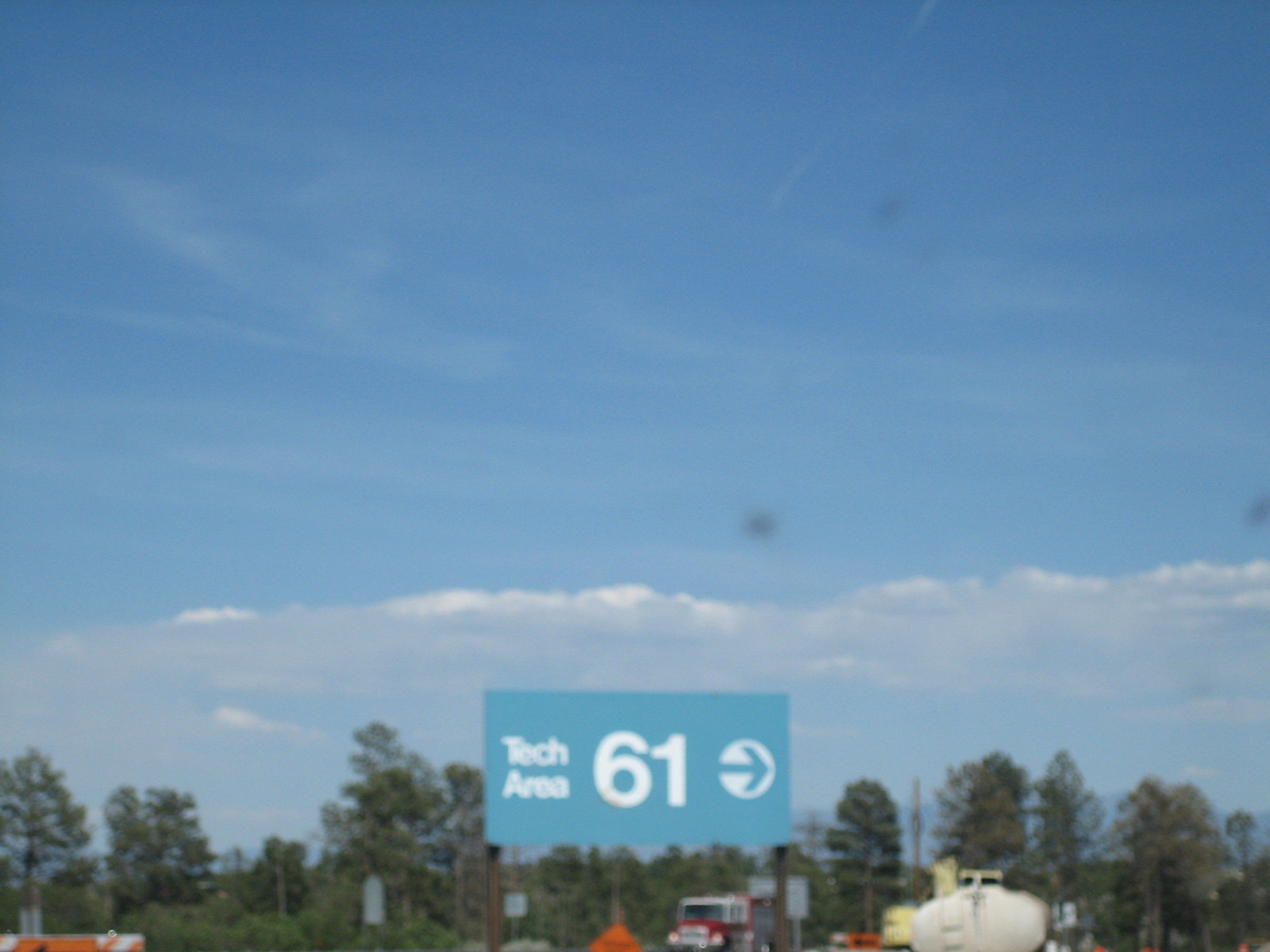Under a clear, light-medium blue sky dotted with a few puffy white clouds, a unique blue sun with intricate tech markings and the number '61' catches the eye. This sun is part of a white circle featuring a prominent blue arrow pointing to the right. The background is lush with dense trees, and scattered below are several work trucks, including what appears to be a cement truck, contributing to a bustling industrial setting amidst nature.